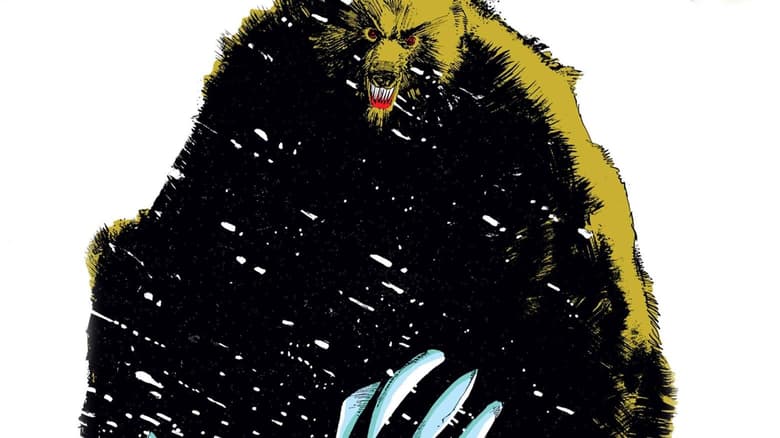This highly stylized drawing, evocative of an adult graphic novel, masterfully depicts a formidable grizzly bear against a stark white backdrop. The bear's menacing visage dominates the image as its head is rendered in a light brownish-yellow hue, cut off just above the eyes, which are fiercely focused downward in a concentrated glare. The eyes themselves are striking, with fiery red centers encircled by yellow and further outlined in black. The bear's gaping mouth reveals sharp, snarling teeth beneath a black-tipped nose. 

The artwork skillfully transitions from detailed coloration at the head, flowing into a light brown-green along the bear's back and shoulder on the right side. The rest of the bear's massive, imposing body descends into an abyssal jet black void, conveying an aura of shadowy dread. This inky darkness is punctuated by what appears to be streaks of snow, cascading diagonally from the top left to the bottom right.

Emerging from this void at the bottom of the image, four large silver claws extend menacingly toward the viewer, highlighting the bear's sheer power and threat. The overall composition, characterized by its deep contrasts and sinister mood, ensures the bear's intimidating presence is felt by all who gaze upon it.